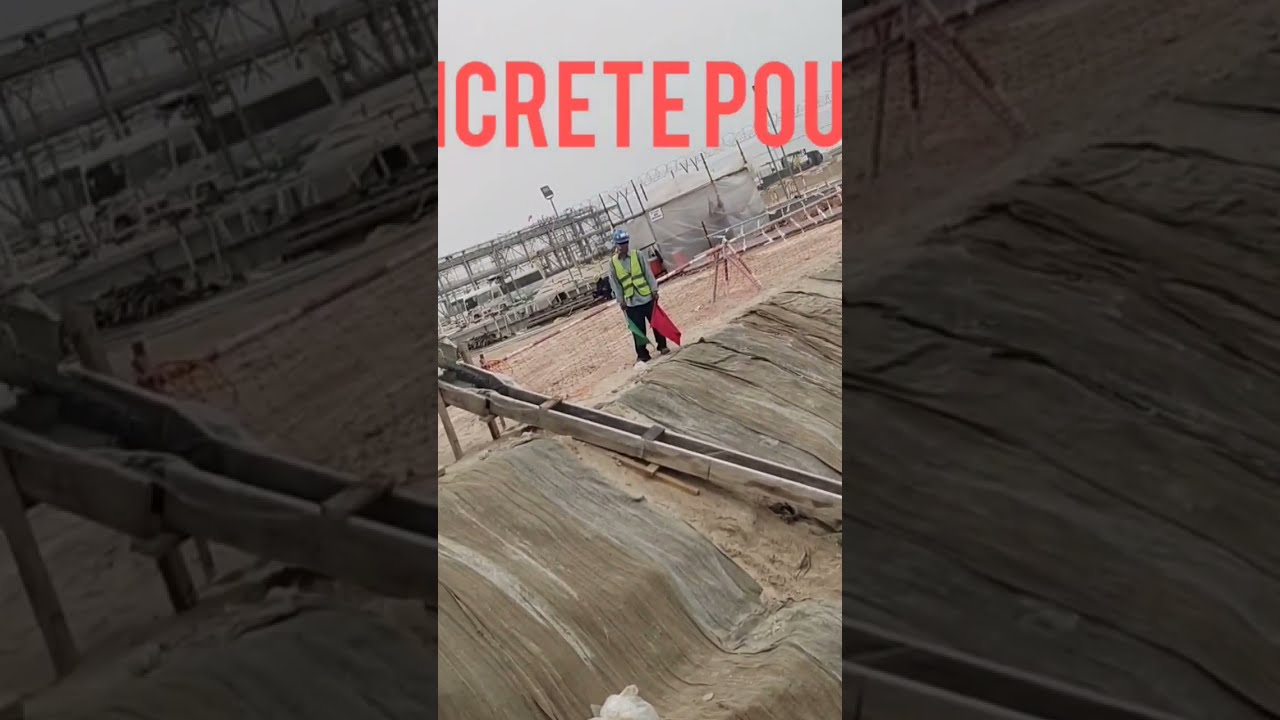This image captures a construction site scene with a man at its center, slightly tilted to the left. He is dressed in a fluorescent lime green safety vest with gray stripes and blue jeans, and he wears a blue construction helmet. In his hands, he holds a red flag in his left hand and a green flag in his right. The background is a mix of gray and tan hues characteristic of a construction site, featuring concrete barriers, a dirt ground, and various materials typical of such an environment. Behind him, a red and white safety fence encloses the area. There appears to be an apparatus, likely for pouring liquid concrete, and possibly a concrete slide coming from a truck at the bottom of the image. An overcast sky adds to the scene's muted color palette. At the top center, partially visible text in capital orange letters reads "I-C-R-E-T-E-P-O-U."